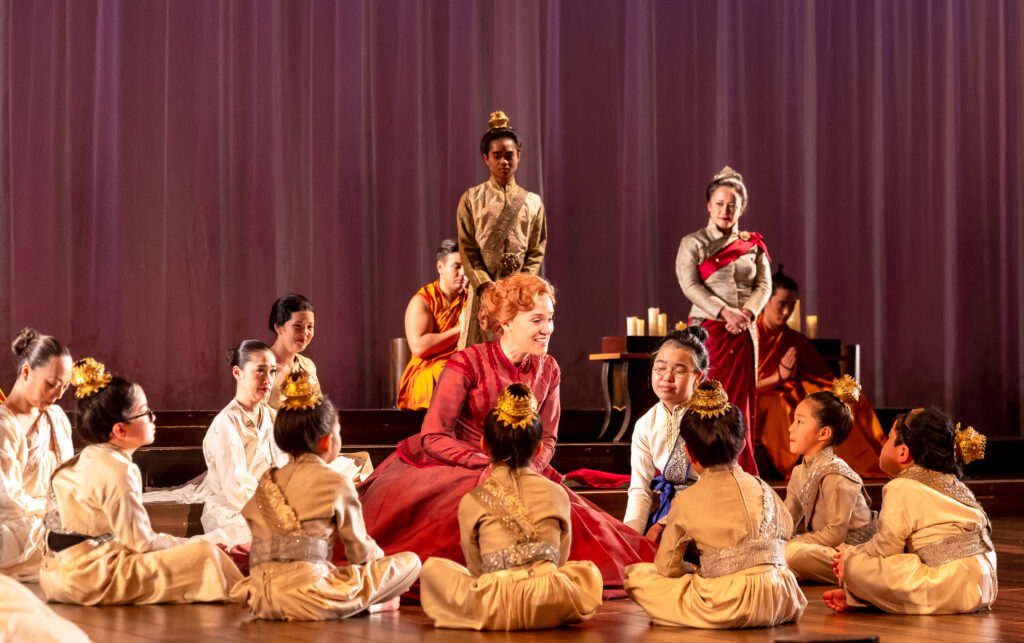The image is a vivid color photograph depicting a scene from a performance of "The King and I." At the center of the stage, long theater curtains serve as a backdrop. A red-haired woman, appearing Caucasian and dressed in a flowing red gown, sits on the floor. She seems to be engaging with a circle of young Asian girls around her, who are all attentively listening and displaying expressions of enjoyment. These girls are dressed in vintage, champagne-colored oriental-style costumes, featuring silvery sashes and adorned with gold brocade or bun holders in their hair that is styled in buns. Behind them, several adults in lighter-colored dresses are visible; they lack the ornate hair accessories of the children. Also in the background, there are a few men, seemingly in orange monk robes, along with tables set with candles. Notably, there is a figure who might be portraying the King, standing reverently with hands clasped in prayer, accompanied by another individual also in a prayerful pose. This setting encapsulates a moment of cultural storytelling or instruction in the theatrical performance.